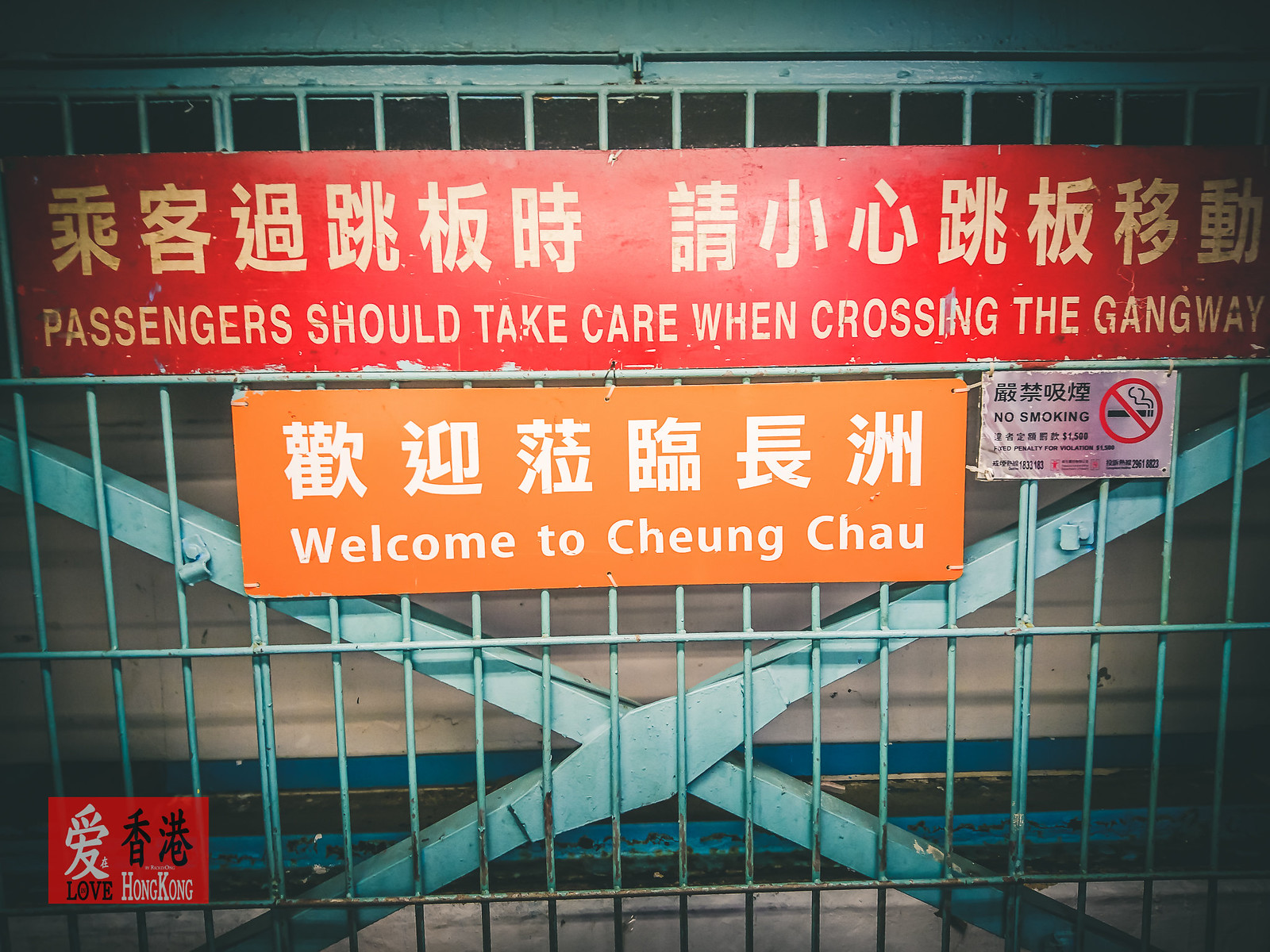This image captures a metal gate or fence situated in Asia, likely Hong Kong, given the visible watermark "Love Hong Kong" in the bottom left corner. The fence is painted in a grayish-blue or light blue hue, with vertical and horizontal bars, and features two large blue bars crossing each other behind it. Prominently displayed at the top of the fence are two signs with both Chinese characters and English translations. The red sign reads, "Passengers should take care when crossing the gangway," and the orange sign below it states, "Welcome to Cheung Chau." To the right of these signs is a white "No Smoking" sign, which includes a pictogram of a cigarette crossed out with a red line. Overall, the image conveys a sense of welcoming caution, with clear multilingual signage ensuring important information is accessible to all.